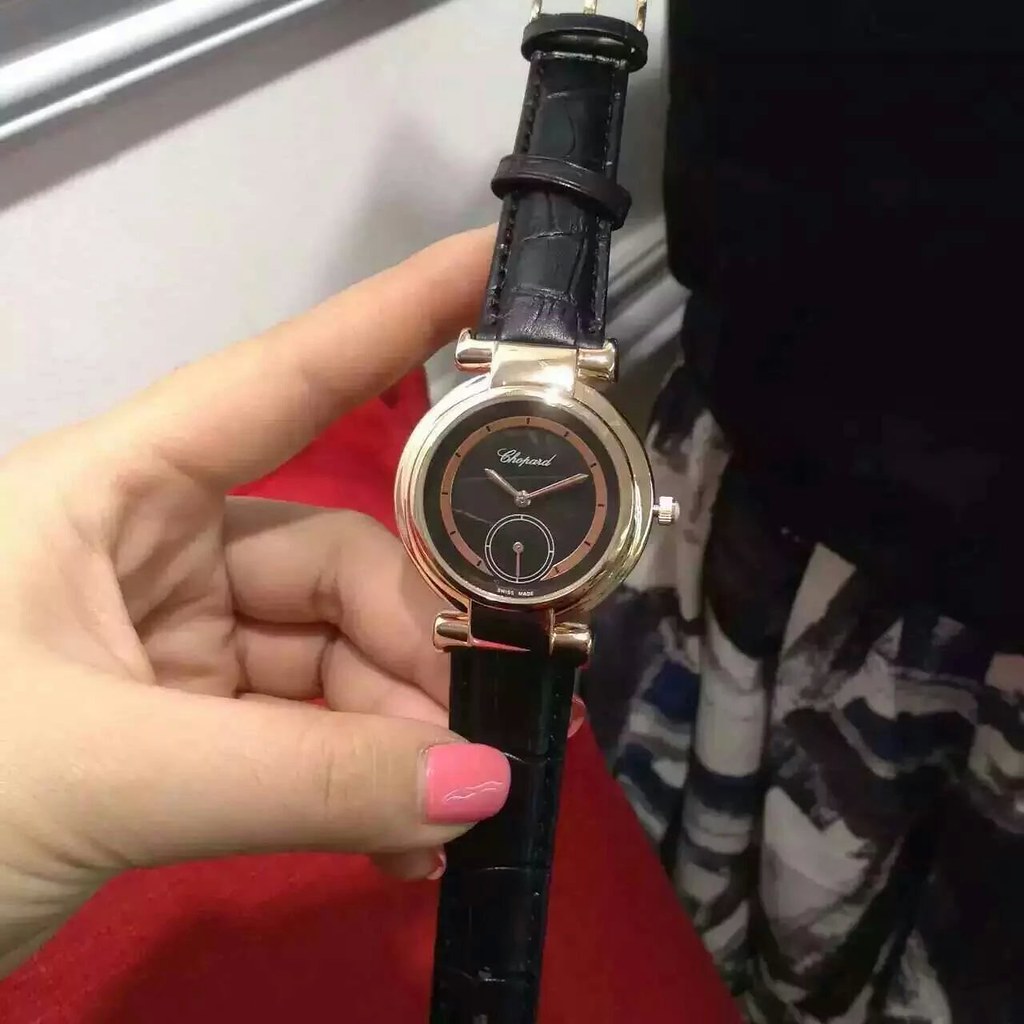In this close-up photograph, a woman's left hand, adorned with pink nail polish, holds a sophisticated wristwatch. Her thumb supports the lower black leather strap—styled to resemble alligator skin—while her index finger steadies the upper strap. The watch, encased in a metallic gold housing, features a black face framed by a medium-sized brownish ring marked with dash lines for the hours, without numerals. The time reads approximately 10:11 or 10:12, shown by two gold hands, and the cursive logo "Chopard" is prominently displayed at the top of the watch face. An additional inset dial sits at the bottom center, possibly a chronograph or second hand, with a single hand pointing to the right. There is one wind-up crown on the right side of the watch. In the background, a red pill and a camo-patterned white and gray blanket are visible, alongside a black object in the top right corner, suggesting the setting could be a transport vehicle such as a bus, train, or airplane.